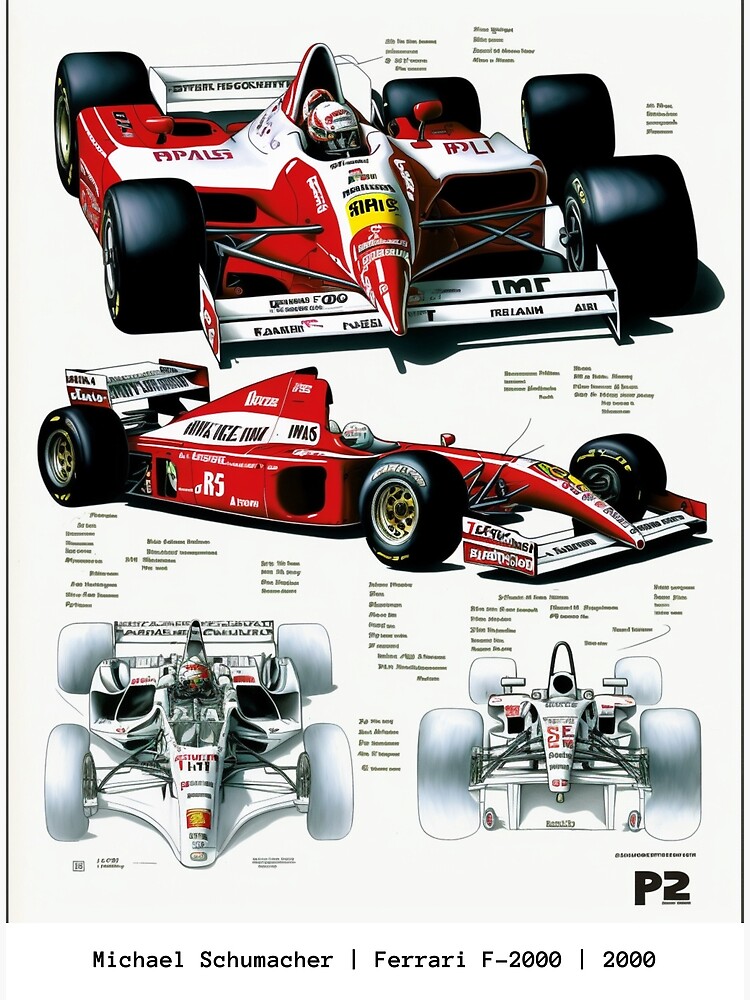The illustrated image features detailed renderings of Michael Schumacher's Ferrari F2000, a renowned Formula One car from the year 2000. There are five distinct views of this Indy-style race car. Four of these views depict the car from different angles: the topmost illustrations showcase a front view at a slight three-quarter angle, prominently featuring the red and white livery with numerous sponsor logos. Below that, another three-quarter side view allows a better look at the car's pointed nose and tail sections. Further down, two smaller, slightly faded out drawings present a direct front view on the left and a rear view on the right. The Ferrari F2000, with its characteristic flat profile and black tires, is optimized for excellent maneuverability and reduced wind resistance. The bottom of the image clearly identifies the car as belonging to the legendary Michael Schumacher, with inscriptions reading "Michael Schumacher Ferrari F2000" and "2000." Additional text, including a "P2" marking at the bottom right corner, suggests this image could be part of an informational poster.